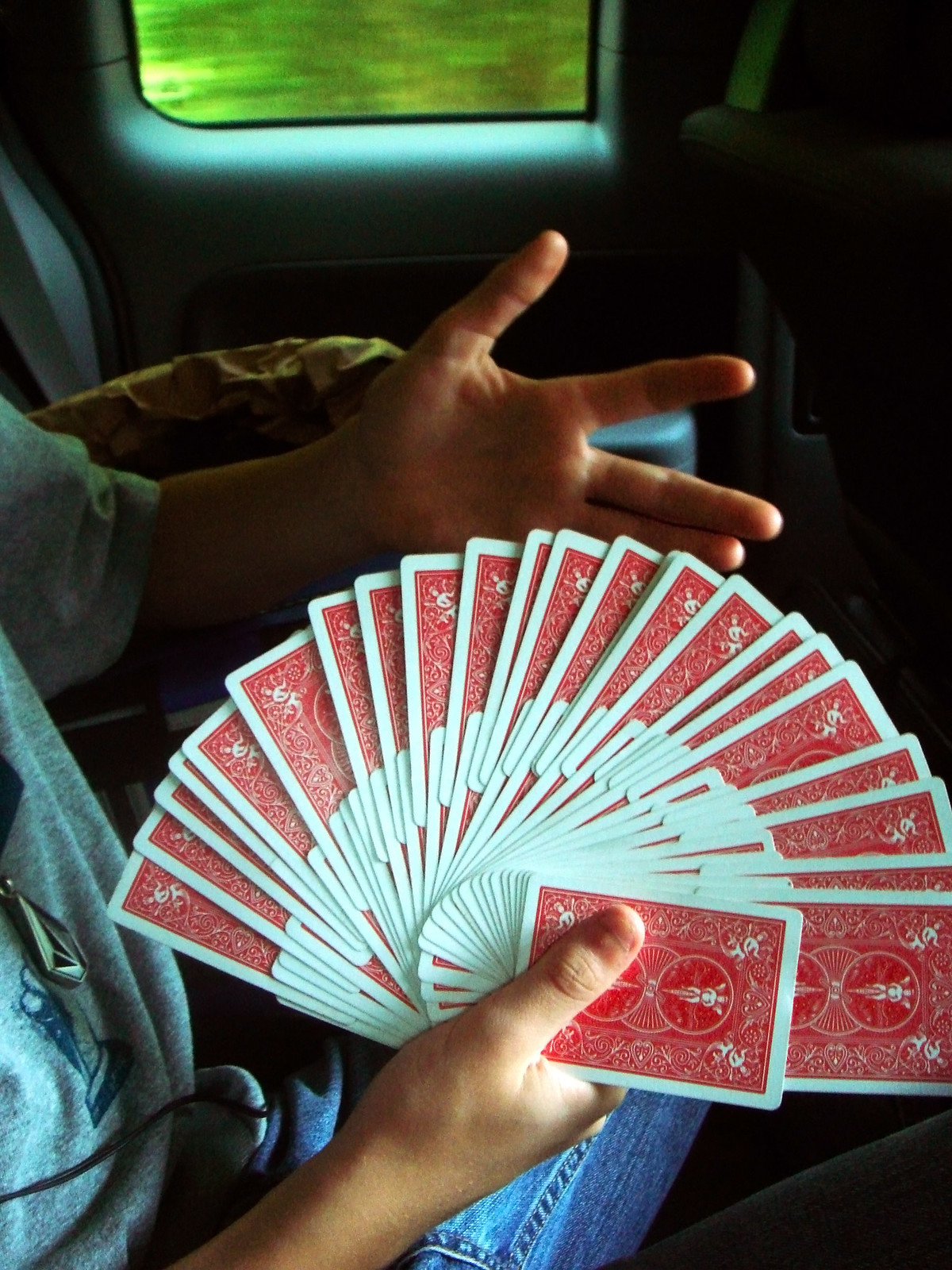In the photograph, a person is seated in what appears to be a vehicle's backseat, possibly a car, bus, or train, given the visible seatbelt apparatus and passenger seat in front of them. They hold a fan of playing cards in their right hand. Interestingly, the fan is doubled, as if a second row of cards has been carefully inserted between those in the first fan. Their left hand is positioned behind the fan, palm exposed and facing the camera, seemingly emphasizing the intricate card display. The person is attired in a gray t-shirt and blue jeans, with a silver necklace around their neck. The view outside the window shows blurred greenery, suggesting rapid movement. Beside them, a yellow item, potentially a bag or jacket, lies crumpled on the seat. The focus remains primarily on the hands, cards, and part of the person's torso.